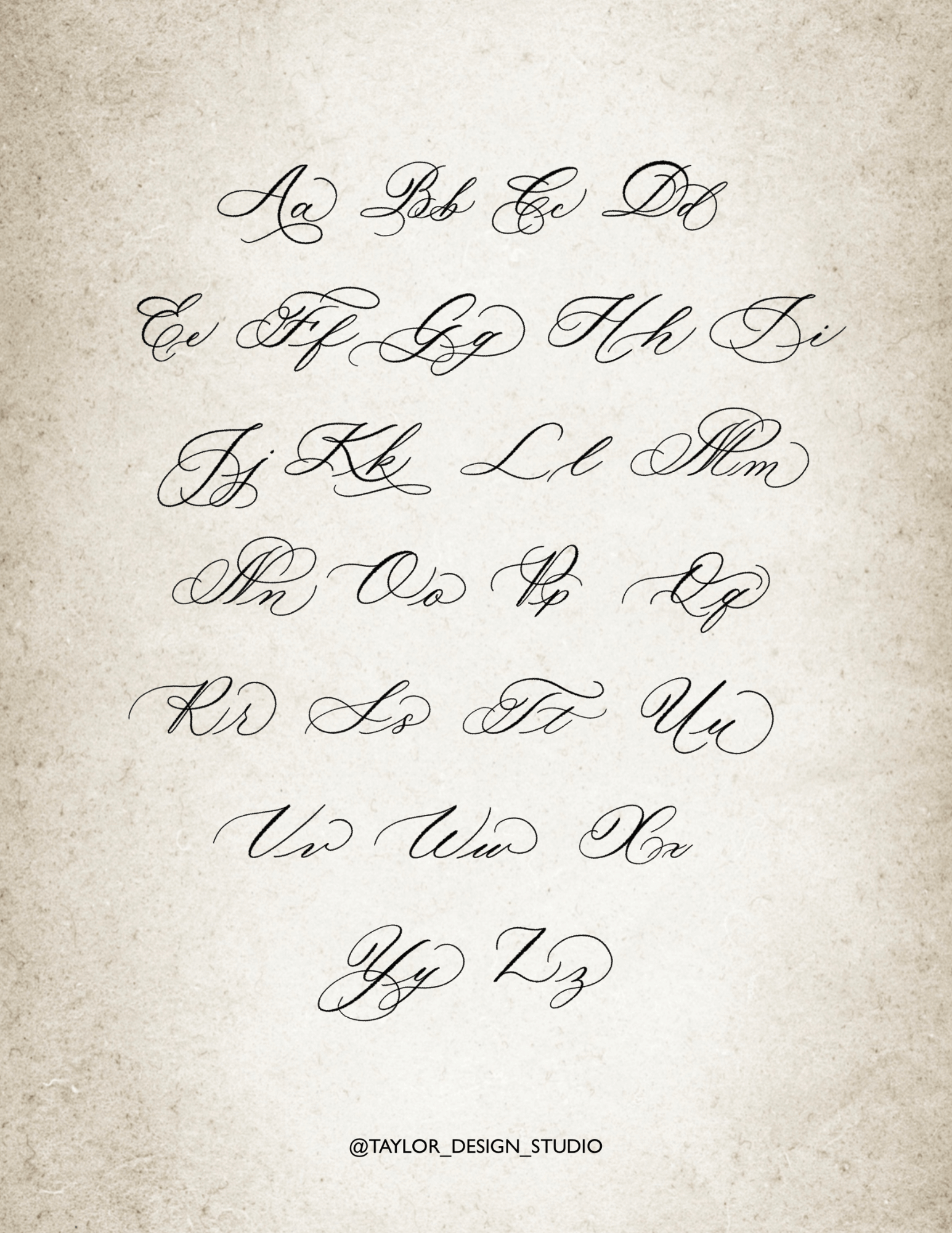This image depicts an example sheet of the entire alphabet in both uppercase and lowercase cursive, presented in a vintage style akin to old-timey textured paper reminiscent of the Declaration of Independence. The background is predominantly light gray with subtle black flecks, and the composition is set within a vertically-oriented rectangular frame. The alphabet is meticulously arranged in seven centered horizontal rows, each pairing an uppercase letter with its corresponding lowercase letter in an ornate, heavily curved cursive style. The sequence follows standard alphabetical order: 
- The first row displays A, B, C, D.
- The second row shows E, F, G, H, I.
- The third row has J, K, L, M.
- The fourth row lists N, O, P, Q.
- The fifth row presents R, S, T, U.
- The sixth row contains V, W, X.
- The seventh row features Y, and Z.

At the bottom center of the image, in all capital letters and black text, it reads "AT TAYLOR DESIGN STUDIO" (some versions mention "at Taylor underscore design underscore studio"), completing the clean, elegant look of this digital representation meant to have a vintage stationary appearance.